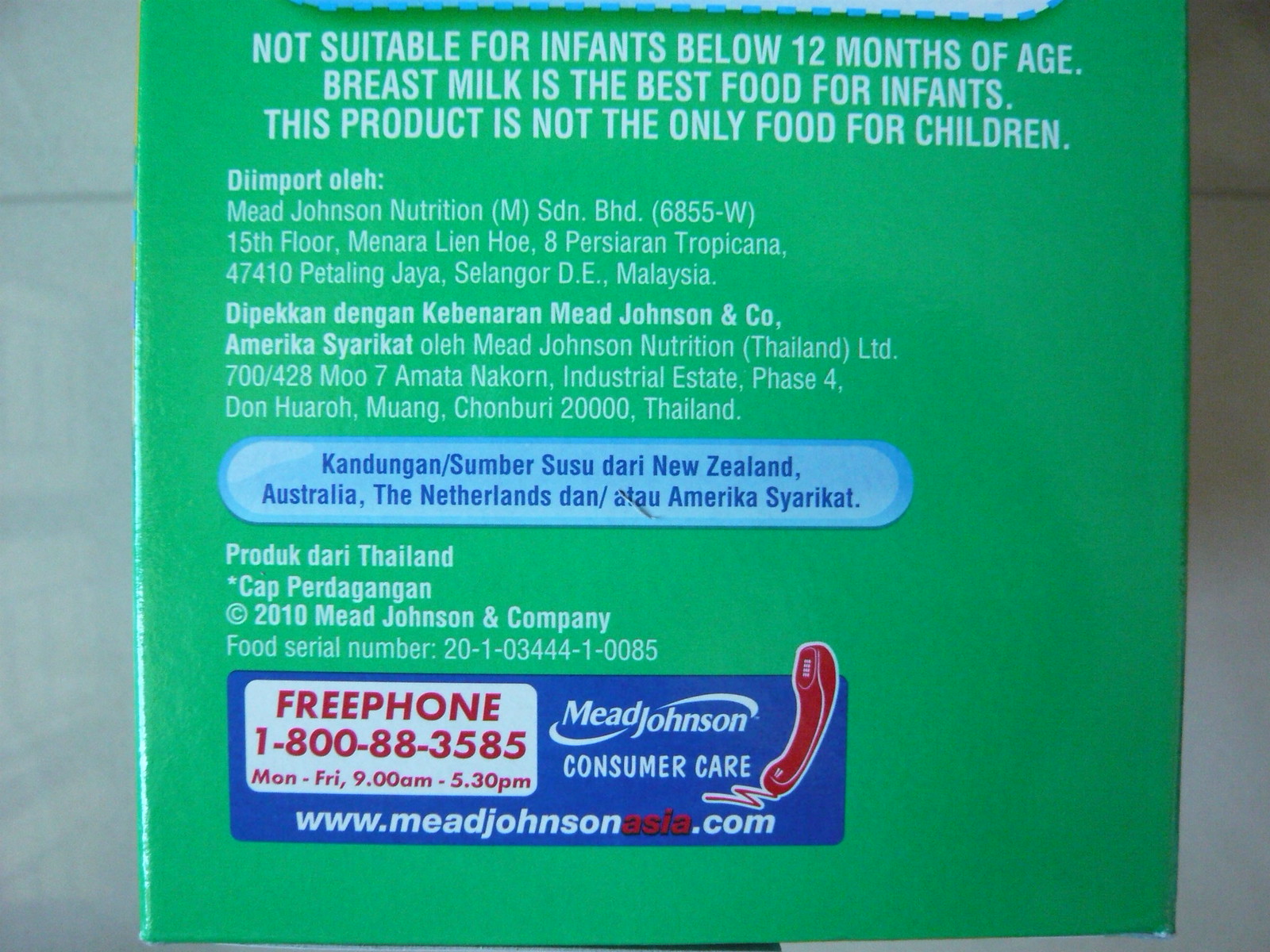This is an indoor photograph of the back of a vividly green product packaging, captured under natural light that enters from the left side of the image. The background is composed of pale grey or white tiles with subtle reflections noticeable on the right side and pale grey grouting lines. The green packaging displays a white line on the left edge, indicating the presence of bright light, while the right side remains in shadow.

The top of the packaging contains a white text warning: "Not suitable for infants below 12 months of age. Breast milk is the best food for infants. This product is not the only food for children." Below this warning, there is information about the head offices of the brand in various locations. A blue pill-shaped icon suggests the product's availability in New Zealand, Australia, the Netherlands, and America. Additionally, the text "Product of Thailand" is displayed in Thai. A blue box at the bottom of the packaging provides details on how to contact the manufacturer's customer care.